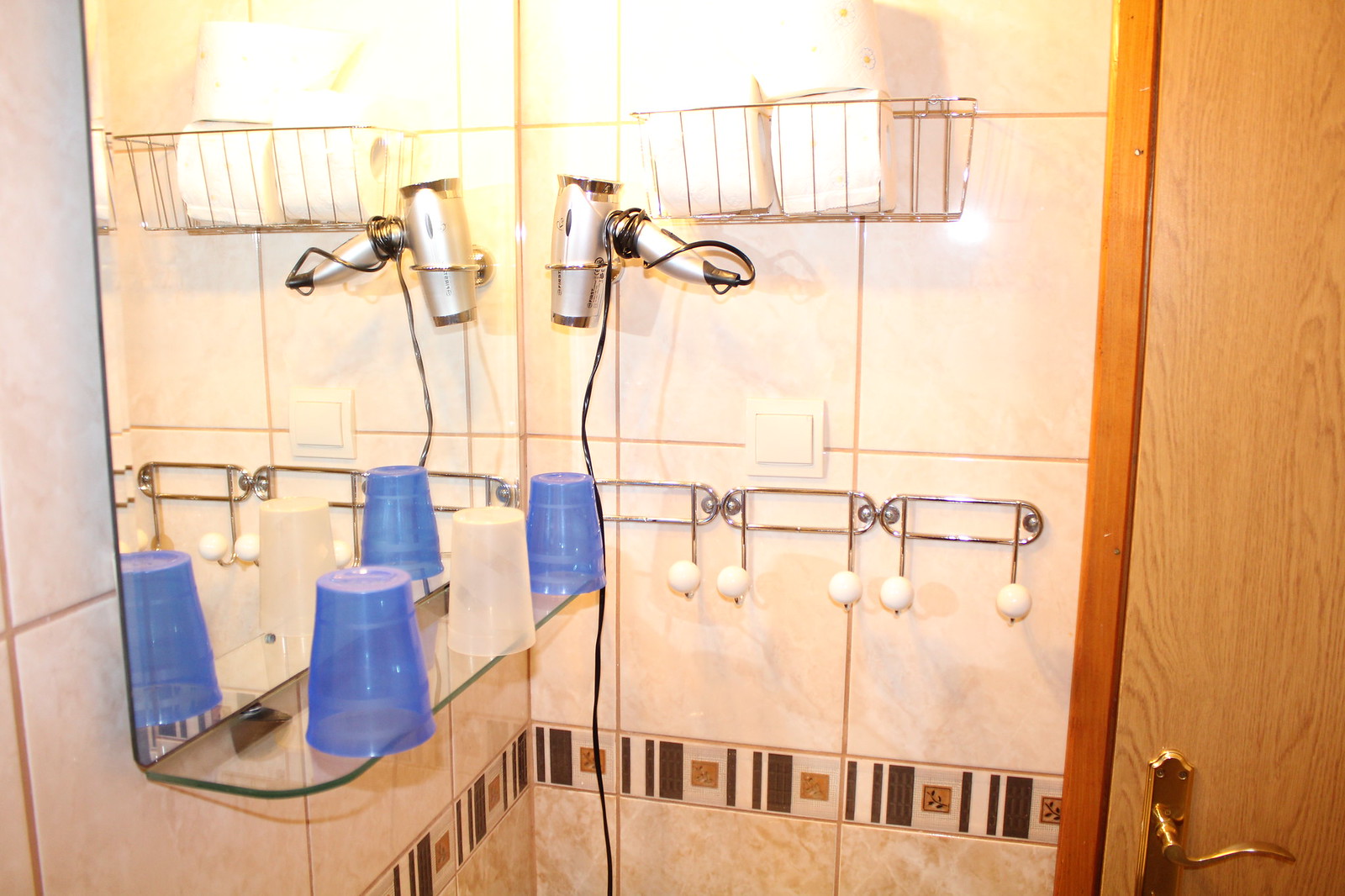The image depicts a detailed view of a bathroom, possibly within a hotel room. The setting features tan tile walls with a distinctive trim of white and gray stripes, interrupted by small brown squares. To the left, a mirror is mounted above a short glass vanity ledge, which holds three upside-down cups—two blue cups on the edges, flanking a clear or white cup in the middle. Above the mirror is a caddy containing towels and toilet paper, with a row of three dual-hook fixtures and a light switch beneath it. A silver blow dryer with a black cord hangs from a hook on the wall. In the foreground to the right, a medium wood-tone door with a gold handle is visible, providing an additional element of warmth and contrast to the scene. The perspective suggests an L-shaped layout, with the corner of the bathroom positioned towards the left side of the image.